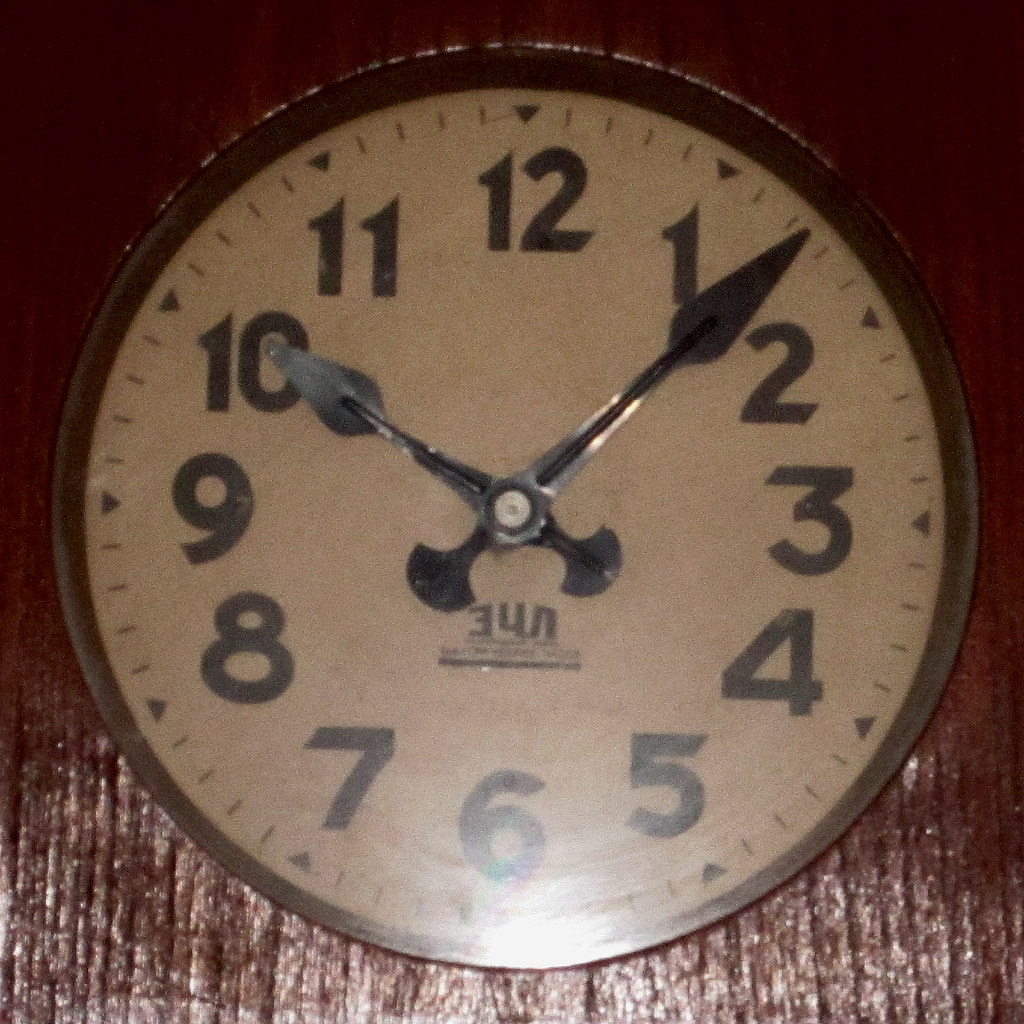The photograph captures an old, circular clock centered on a textured, varnished wooden wall with a noticeable light glare predominantly at the bottom, gradually darkening upwards. The clock reads approximately 10:07 or 10:08, with the small hand on the 10 and the large hand between the 1 and 2. The clock's face is a faded light gray or taupe color, encircled by a black border. The large, bold numbers, possibly in Helvetica font, along with black lines and triangles, clearly mark the hours. The clock hands are metallic black, partially chipped to reveal a silver undertone, giving them a worn appearance. A bolt secures the hands at the center, and beneath them, there are letters that seem to be in a different language, potentially Russian. The photograph has a slightly grainy quality, suggesting it's an older image.